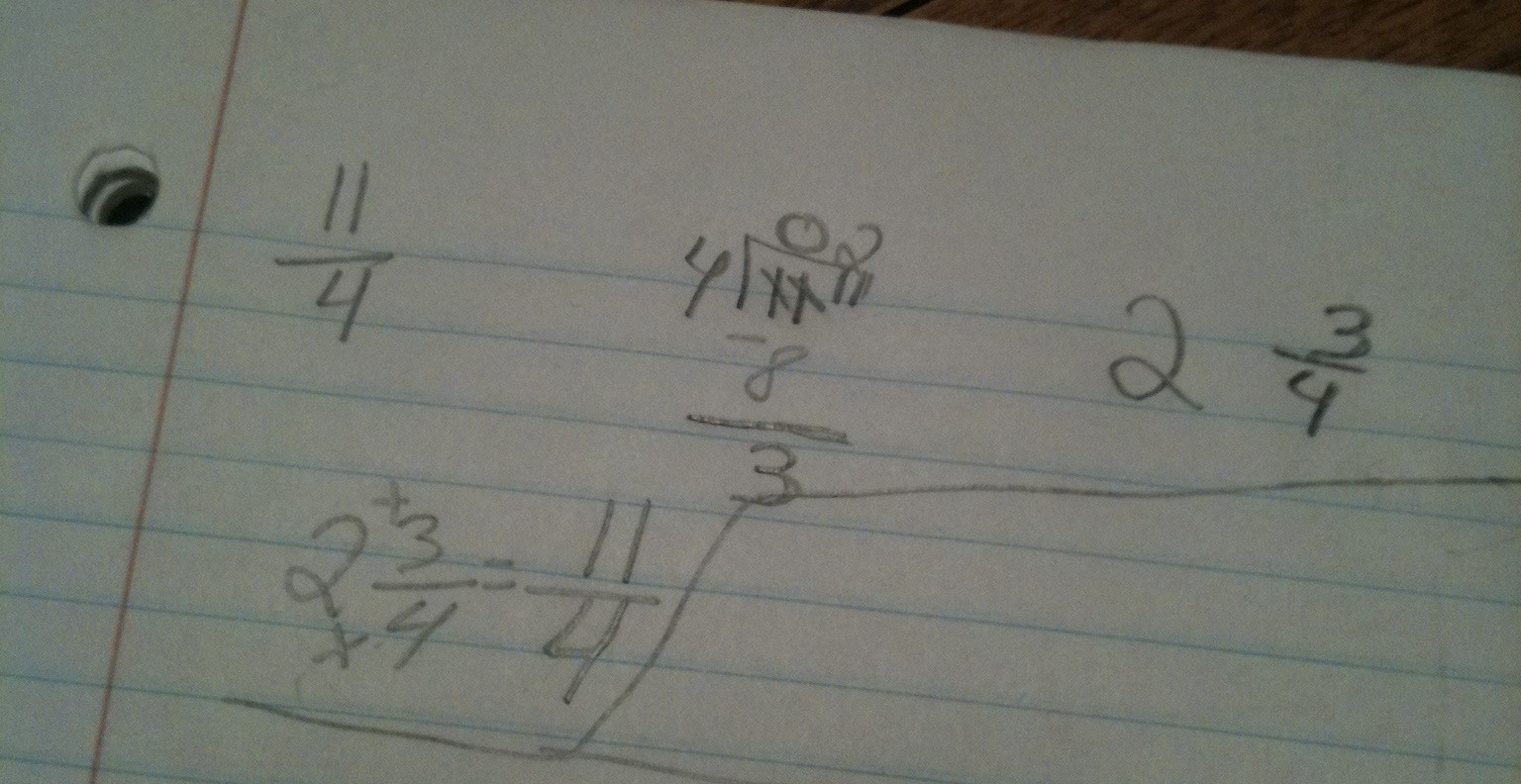A close-up image captures the top left section of a piece of scholastic notebook paper. The paper is lined horizontally with blue lines and features a single binder hole in the upper left corner. Several incomplete math problems are scribbled across the visible portion of the page. On the far left, the fraction "11/4" is noted. The right side shows "2 3/4," and in the center, the fraction "4/11" is worked out with the result “3.” At the bottom left, another problem involving "2 and 3 quarters" is noted, although the corresponding math seems unfinished or incorrectly stated as "11 and a quarter." The image appears to be a snapshot of someone’s math notes, possibly taken during class, as part of homework, or while solving problems ahead of a test.